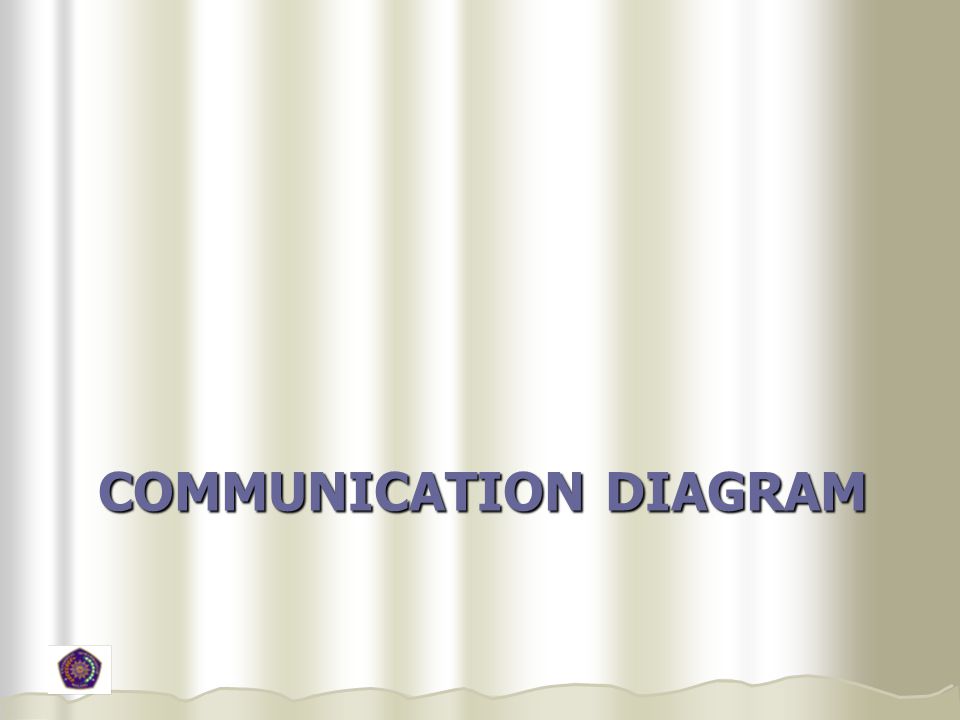The image resembles a PowerPoint slide with a textured background in an off-white, eggshell color meant to imitate drapery with subtle wavy patterns. Positioned towards the bottom half of the slide, the all-caps text "COMMUNICATION DIAGRAM" is prominently displayed, rendered in a mauve or aqua color. In the bottom left corner, there's a small pentagon-shaped logo featuring colors like purple, pink, orange, blue, and mint green, with possibly a central design resembling either a sun or wheel. A very faint gray line extends upward from the logo to the top of the image, adding to its minimalist design.